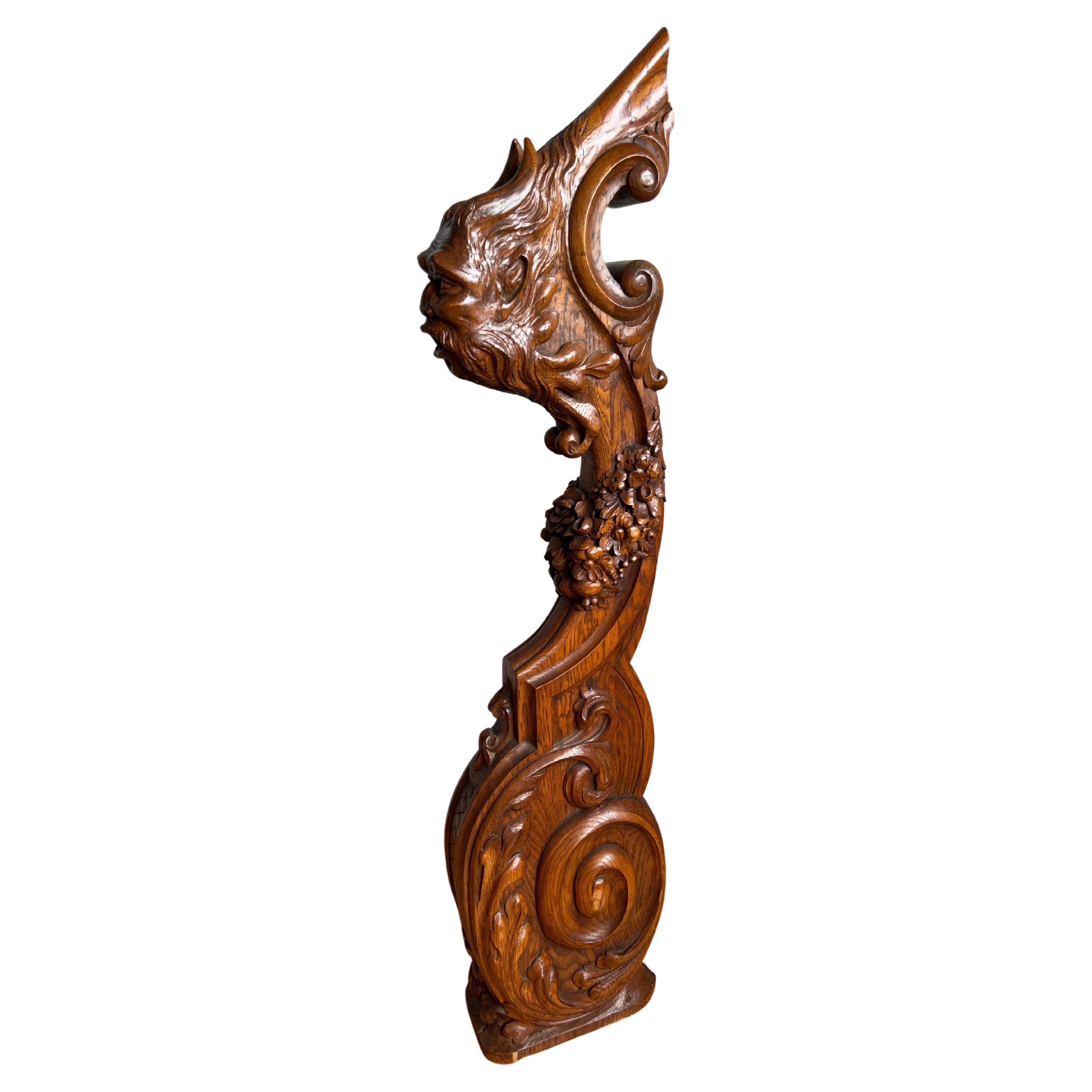The detailed description of the elaborate wooden item in the photograph is as follows:

The image presents an ornately carved wooden piece that seems to be an integral part of furniture or perhaps a railing of a stairway, potentially the end piece. The piece is crafted from dark wood and exhibits exceptional detail and artistry. At the top of this sculpture, there is a meticulously carved face resembling an old man or a mythological figure, like a Viking or Poseidon. The face features long flowing hair and a beard, with an expression that appears somewhat concerned or upset, with an open mouth. The hair is intricately detailed, giving a sense of movement as though blown by the wind, reminiscent of figures carved into the mastheads of ships.

The design flows downward in an S shape, transitioning into a series of spiraling curves. Along this descent, the piece is adorned with intricate patterns, including fine floral carvings and plant-based swirls. These elements are delicately executed, with smaller flowers interspersed among the floral and scroll designs. The base of the wooden piece is thicker and sturdier, continuing the decorative motif with additional floral and natural elements that enhance its ornate appearance. Overall, the sculpture is a testament to skilled craftsmanship, combining both utility and aesthetic appeal, making it a standout artistic wooden component.